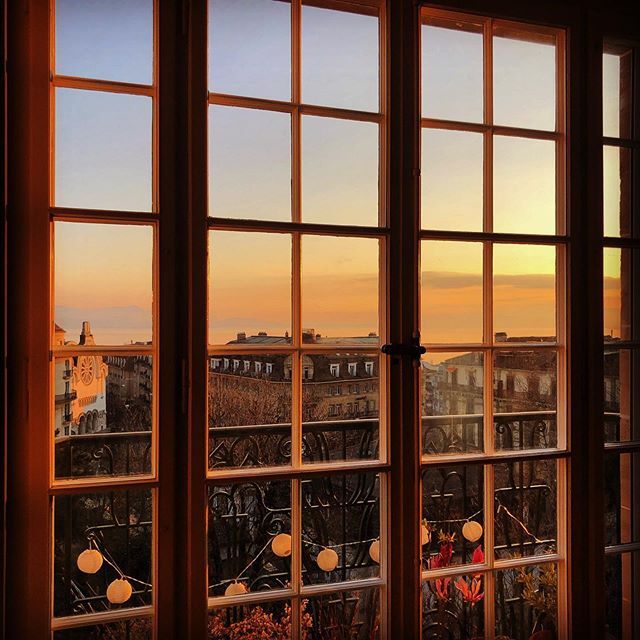This photograph captures a serene cityscape at either sunrise or sunset, with warm, muted tones of brown, orange, yellow, red, and hints of light blue and pink adorning the sky. The vantage point is from inside, looking out through beautiful paned French doors. Beyond the doors lies a black metal wrought iron balcony, decorated with plants with red leaves and small decorative lanterns with white round globes. This intimate outdoor space overlooks a European city skyline, comprised of large, squat buildings with large windows, reminiscent of those found in Germany or France. In the distance, a body of water is faintly visible, adding to the tranquility of the scene. The soft lighting and band of cloudiness along the horizon enhance the overall ambiance, creating a picturesque and inviting view.